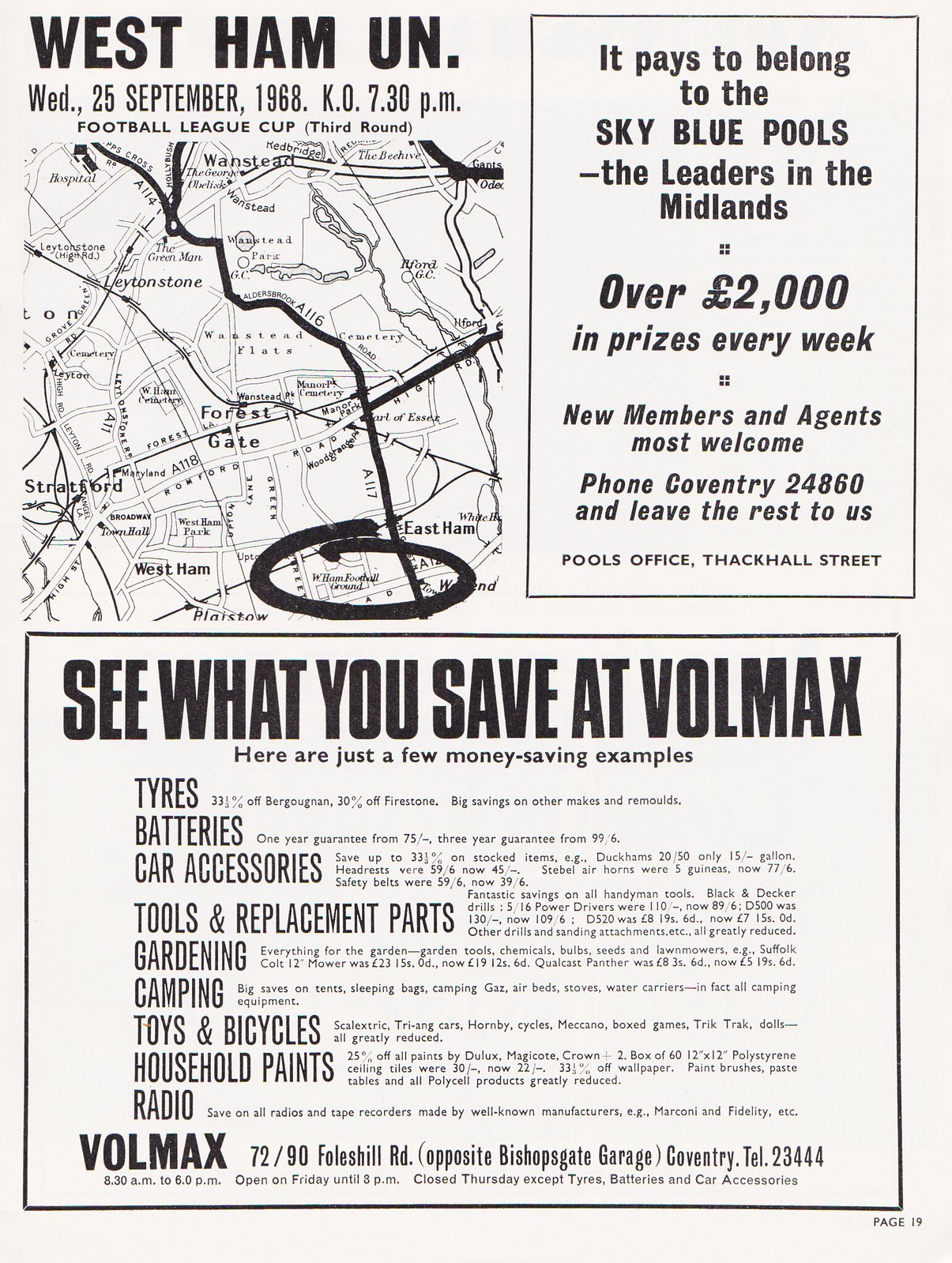This image is a scanned page from a magazine or newspaper, primarily using black text on a white background. At the top left, it prominently displays the event details: "West Ham United, Wednesday, 25th September 1968, K.O. 7.30 PM, Football League Cup Third Round." Adjacent to this text, there's a map with a circled area marking the location of the game. The map provides directions for attendees.

In the upper right section of the page, there's a column advertisement for the Sky Blue Pools, asserting their leadership in the Midlands. It promises over 2,000 pounds in prizes every week and invites new members and agents to join. The contact details are provided as "Phone Coventry 24860, and leave the rest to us." The address mentioned is Pools Office, Thickhill Street.

Towards the bottom, another advertisement promotes Volmax with the statement "See what you save at Volmax." It lists money-saving examples including tires, batteries, car accessories, tools and replacement parts, gardening and camping equipment, toys and bicycles, household paints, and radios. The address is specified as "Volmax, 72-90 Foleshill Road, opposite Bishopgate Garage, Coventry," with the contact number "Tel: 23444." At the very bottom right corner of the page, there is a note indicating "Page 19."